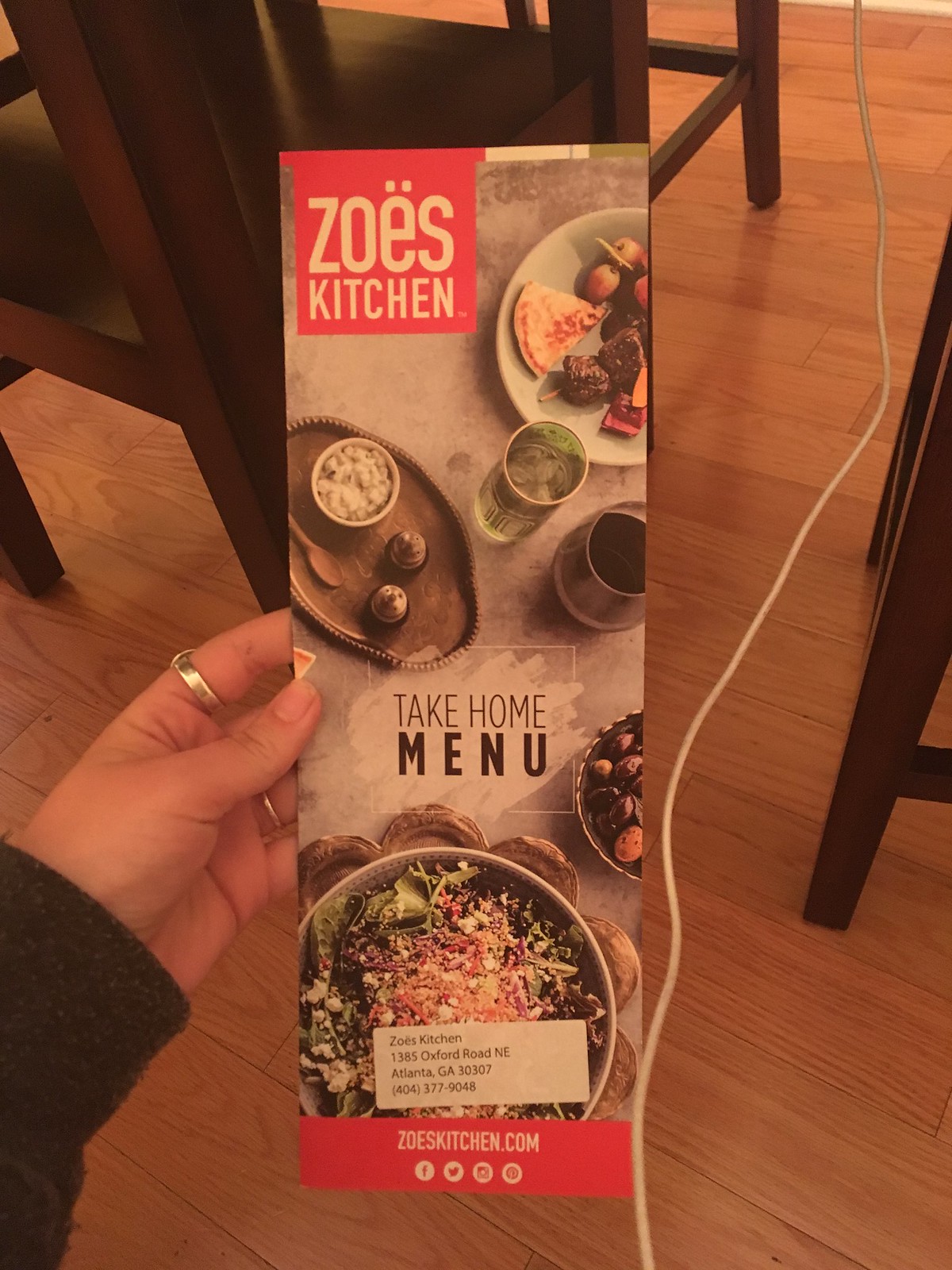In an indoor setting, the photograph captures a vibrant scene inside Zoe's Kitchen restaurant. Prominently featured in the image is a take-home menu held by a woman with a fair-skinned hand, dressed in a gray shirt. The menu is striking with "Zoe's Kitchen" written in bold white letters against a vivid red background. 

At the top left corner of the menu, there are enticing pictures displaying various entrees and drinks. Centrally, the black letters spell out "Take Home Menu." The bottom of the menu repeats the "Zoe's Kitchen" branding in white letters, again set against a red border. Below this, there are logos for social media platforms, including Facebook, X, Instagram, and another unidentified icon.

A wooden floor provides the backdrop, adding a warm, rustic touch to the composition. Notably, a white cord runs diagonally across the floor, stretching from the foreground to the back of the photo. In the upper left section, partial views of brown chair legs suggest nearby seating, enhancing the restaurant's cozy, welcoming atmosphere.